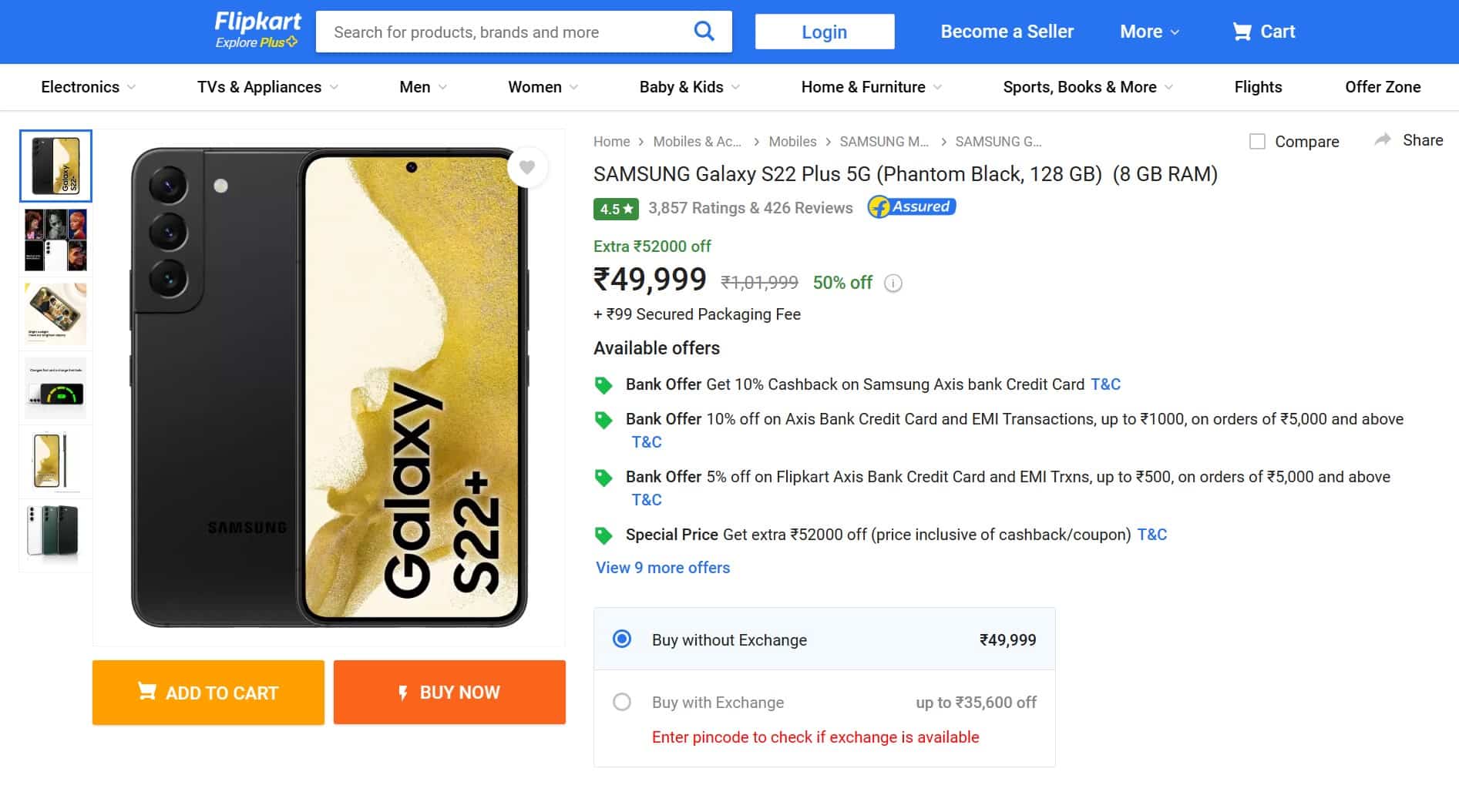This image is a screenshot from the Flipkart website, showcasing a prominent blue banner at the top. The banner features the Flipkart logo alongside the "Explore Plus" tagline, and to the right, there's a search bar with a blue icon within a search box. Adjacent to the search bar are options for logging in, becoming a seller, exploring more options, and viewing the cart.

Below the blue banner is a white navigation bar listing various categories: Electronics, TVs & Appliances, Men, Women, Baby & Kids, Home & Furniture, Sports, Books & More, Flights, and Offers. Each category is arranged from left to right.

Centrally featured is a promotional detail for the Samsung Galaxy S22+ 5G, Phantom Black variant with 128GB storage and 8GB RAM. This product has a rating of 4.5 stars from 3,857 ratings and 426 reviews. There are special promotional details indicating an assured extra ₹2,000 off from an original price of ₹49,999, indicating a 50% discount. Additional features include a "Secured Packaging Fee" option and available offers.

Highlighted offers include:
- A bank offer providing 10% cashback on Samsung Axis Bank credit cards (terms and conditions apply).
- Another bank offer of up to 10% off on Axis Bank credit card EMI transactions, up to ₹1,000 on orders of ₹5,000 and above.
- A separate bank offer gives 5% off on Flipkart Axis Bank Card EMI transactions, up to ₹500, on orders of ₹5,000 and above.
- A special price with an extra ₹2,000 off, included in the cashback/coupon price (terms and conditions apply).
- Additional 9 offers are viewable under specified conditions.

The product can be purchased without exchange for ₹49,999, or with an exchange for up to ₹35,600 off, subject to availability based on the entered pin code.

To the left of the promotional details, there's an image of the Samsung Galaxy S22+, clearly showing its sleek black design with triple camera circles on the top left and a branding inscription that reads "Galaxy S22+." Smaller icons also suggest the phone comes in different colors like white, gray, and black. At the bottom of the image, there are options to add the product to the cart or proceed with a purchase by clicking "Buy Now."